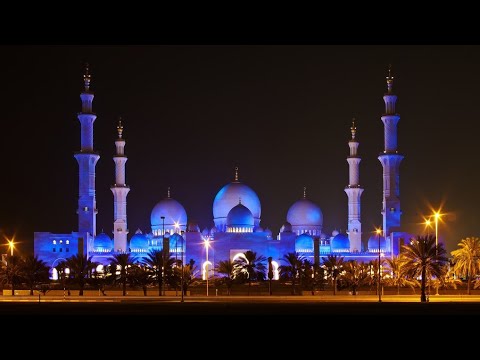This nighttime photograph captures a majestic building that exhibits architectural influences from the Middle East or India, illuminated against a black sky. The structure, which resembles a significant and possibly religious edifice such as a mosque, is accented by a series of lights. The overall blue hue of the building creates a mysterious, almost purplish glow, contrasting with the yellow street lights that cast an amber gleam on the surroundings.

The building itself is an elongated rectangular form with two symmetrically arranged towers on each side—one larger and one smaller. These towers flank a central series of domes: three aligned in a row with another dome positioned in front of them, all of which have round, ball-like roofs capped with sharp pinnacles. The domes appear white under the blue lighting.

In the foreground, rows of palm trees are visible, their bases illuminated by the warm yellow lights. The bottom of the image is engulfed in a thick black area, and tall lampposts on both the far right and left edges shed further yellow and orange star-like points of light onto the scene. The night sky remains a solid, starless black, adding to the dramatic effect of the brightly lit structure against the darkness.